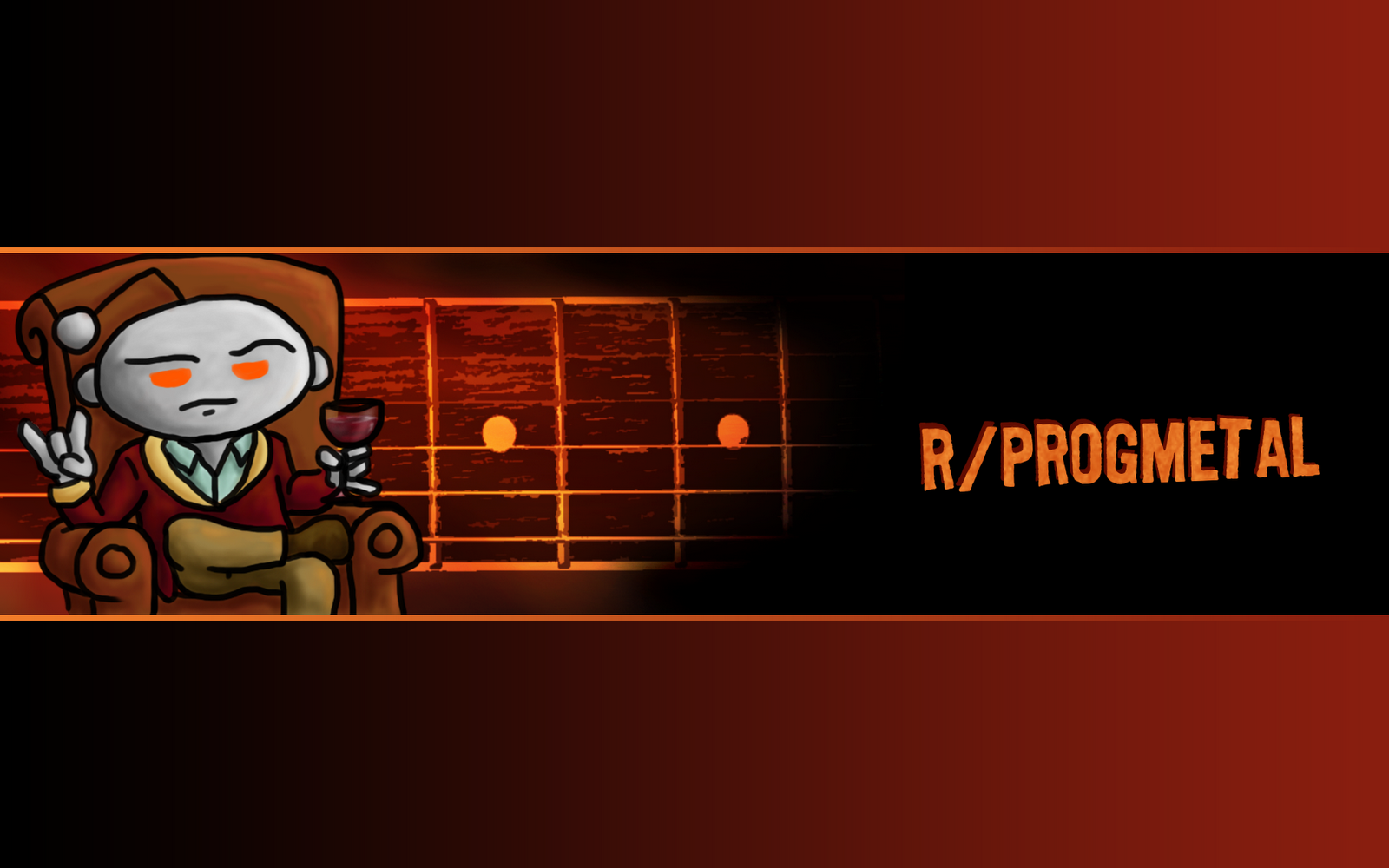The header image for the r/progmetal subreddit features a custom Snoo avatar on the left. The Snoo is dressed in a luxurious smoking jacket and is comfortably seated in a reclining chair. In one hand, the Snoo holds a glass of wine, exuding an air of sophistication. The other hand is raised, displaying the iconic devil horn symbol, commonly associated with metal music fans. To the right of the Snoo, the text "r/progmetal" is prominently displayed. Progressive metal, or prog metal, is a subgenre of heavy metal music, renowned for its complex structures and intricate instrumentation. This subreddit serves as a vibrant community for enthusiasts who enjoy listening to, discussing, and sometimes passionately debating the merits of prog metal. While the fanbase can be fiercely devoted and occasionally elitist, the forum remains a haven for all who share a love for this innovative and dynamic genre.